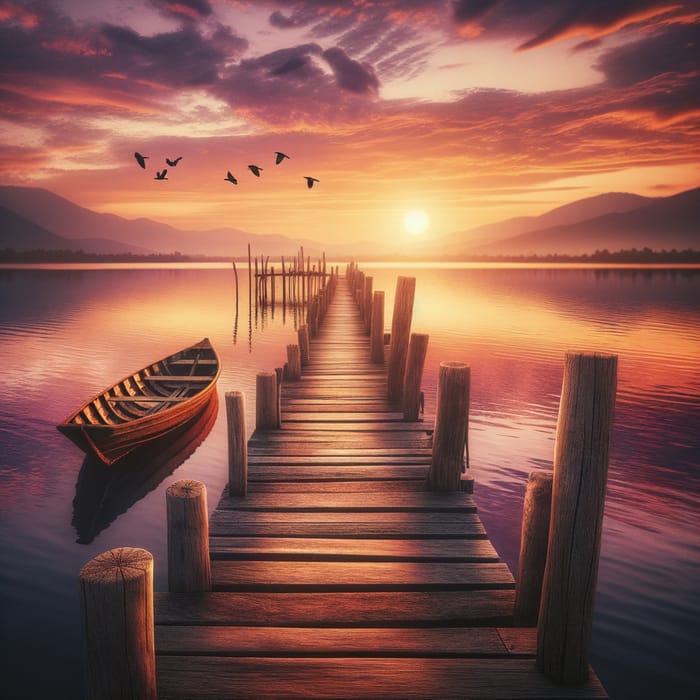The painting depicts a serene lakeside scene at sunset. In the foreground, there is a wooden pier extending out into the tranquil waters, composed of light and dark brown wooden slats and supported by cylindrical pillars on both sides that jettison from the water. The pier snakes into the distance and curves to the left, emphasizing a homely, hand-constructed appearance. To the left of the pier floats a wooden canoe, detailed with supportive wooden planks and cross boards for seating, painted in brownish-red hues with a hint of orange. 

The sky is ablaze with the colors of a setting sun, predominantly featuring orange hues with pink and reddish streaks, while dark clouds cover portions of the left and right sides. The sun itself is positioned just right of center, casting vibrant reflections of gold, purple, and dark-gray-black onto the water below. Above the mountains on the horizon, painted in a purple hue, a flock of seven birds, represented as black silhouettes with outspread wings, soars towards the sun from the left side of the canvas. These birds are grouped into two clusters, adding a sense of movement to the tranquil setting.

The lake’s water mirrors the sky’s kaleidoscope of colors, transitioning from a dark purple to a more vibrant violet with streaks of red near the pier, creating a serene yet vivid interplay of reflections. In the background, the rolling mountains and a distant shoreline lined with tiny, silhouetted trees contribute to the peaceful, reflective mood of the artwork. The entire scene exudes a picturesque, harmonious blend of natural elements, making it a compelling display of sunset beauty.